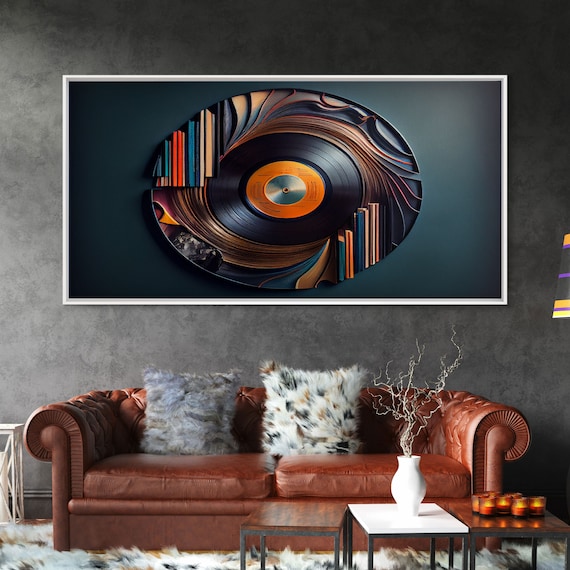This photograph depicts a cozy room with a dark gray wall serving as a backdrop. Dominating the wall is a large rectangular painting framed in white, which features a dark teal background. Central to the artwork is an elliptical shape that closely resembles a warped CD, with a shiny black exterior, an orange interior label, and seemingly melted edges.

Beneath this painting sits a brown leather sofa adorned with two fuzzy pillows. One pillow is gray, while the second is white, spotted with light brown and black. In front of the sofa are three small tables, one of which holds a white plant pot with dry branches. Another table hosts several lit votive candles, adding a warm glow to the scene. The texture of the pillows appears to match the rug that surrounds the seating area, contributing to the room's overall inviting atmosphere.